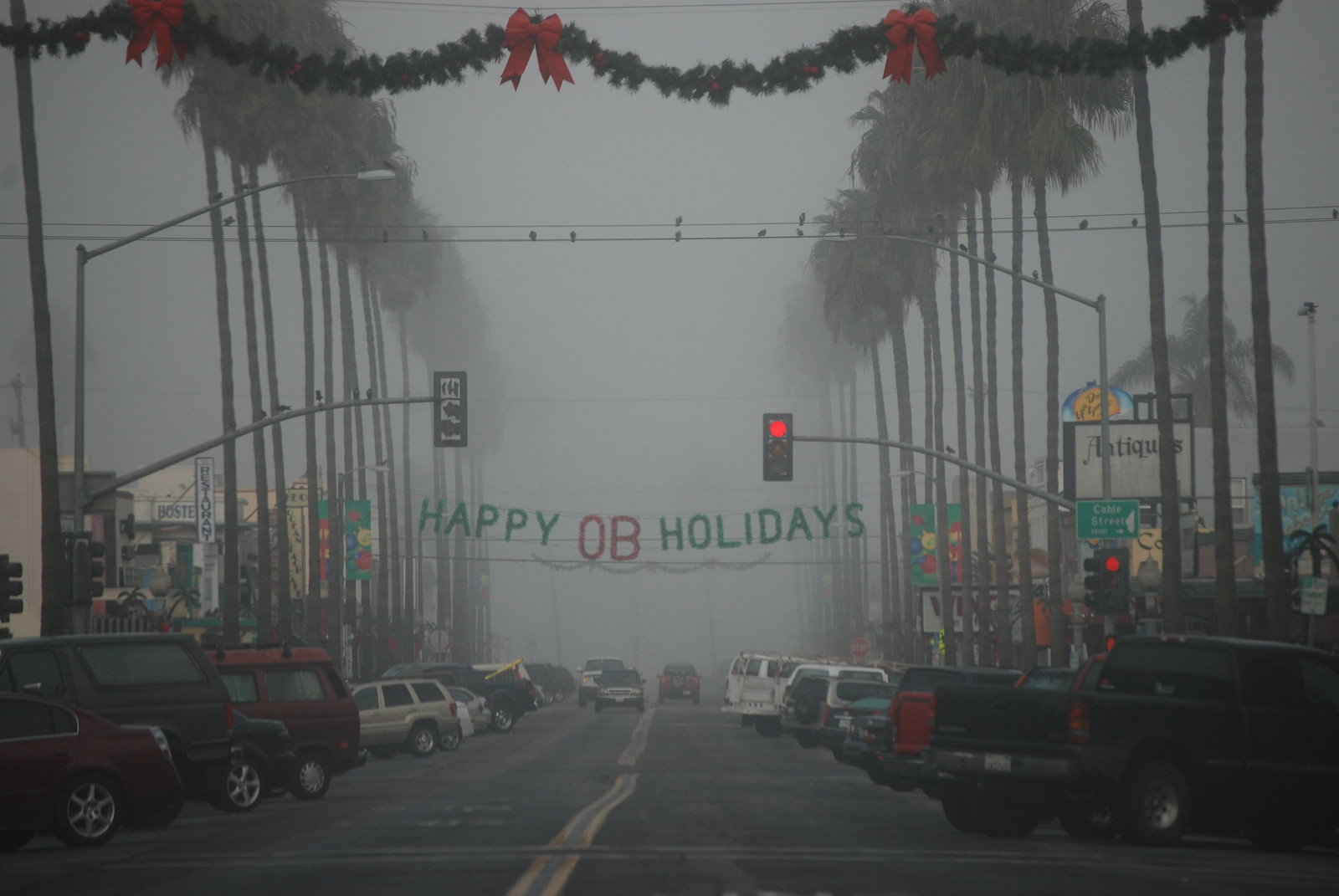The image depicts a very foggy, overcast day on a street lined with tall palm trees, which are about four to five stories high. Cars are parked diagonally on both sides of the road, and a few vehicles are driving down the center, separated by a double yellow line. A prominent festive decoration spans horizontally across the top of the image: a holiday wreath adorned with red bows and ribbons. Just below this wreath is a stoplight that is currently red. In the middle of the image hangs a green sign that reads "Happy Holidays." The foggy weather significantly obscures the background, creating a dull gray atmosphere. Storefronts line both sides of the road, including one with a large white sign that reads "ANTIQUES." Overall, the scene is gloomy yet festive, illuminated by natural light that struggles to penetrate the heavy fog.